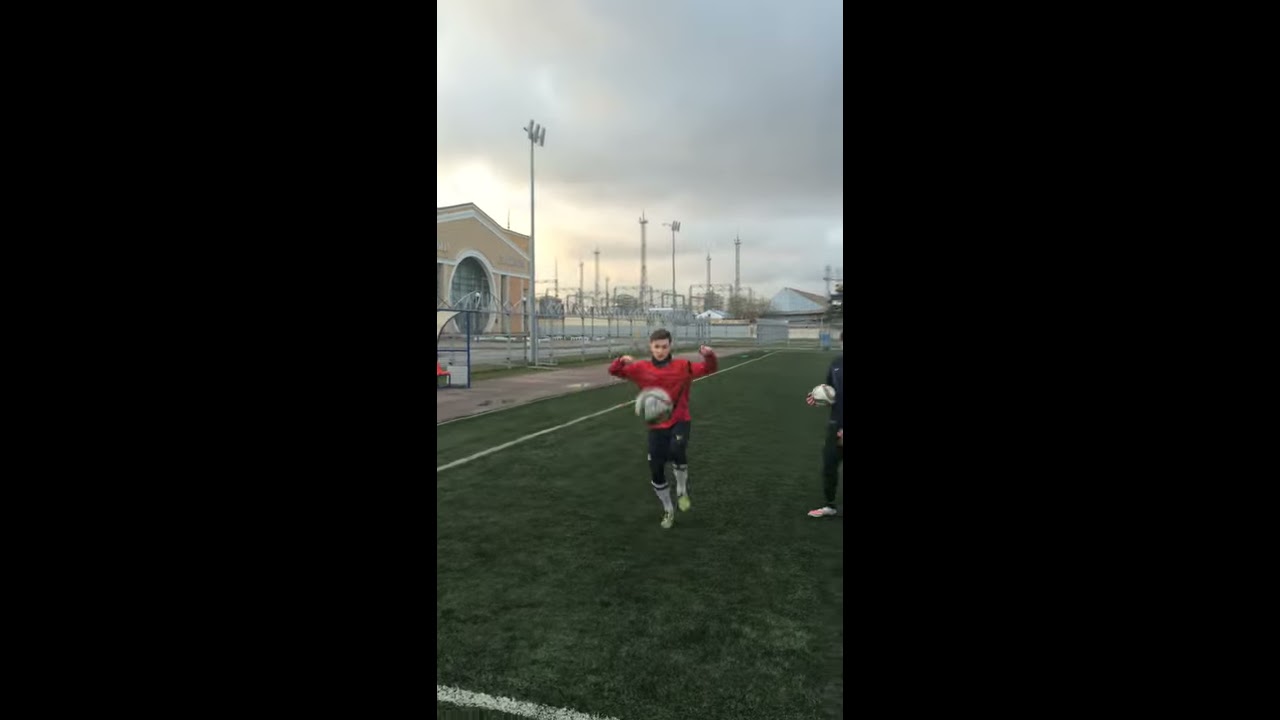This outdoor photograph captures an overcast, dreary day on a grassy soccer field, the white boundary lines clearly visible. At the center, a person dressed in a red long-sleeve shirt, black pants, and white knee-high socks has just kicked or is about to kick a ball that is suspended in mid-air in front of them, their knee raised. To the right of the central figure, another person, likely a coach, stands partially out of the frame, dressed in dark clothing and holding another white ball. In the background, a long fence runs horizontally across the scene, behind which stands a beige brick building with white trim. Tall floodlights tower over the field, completing the somewhat gloomy atmosphere as the sky looms gray with potential rain.